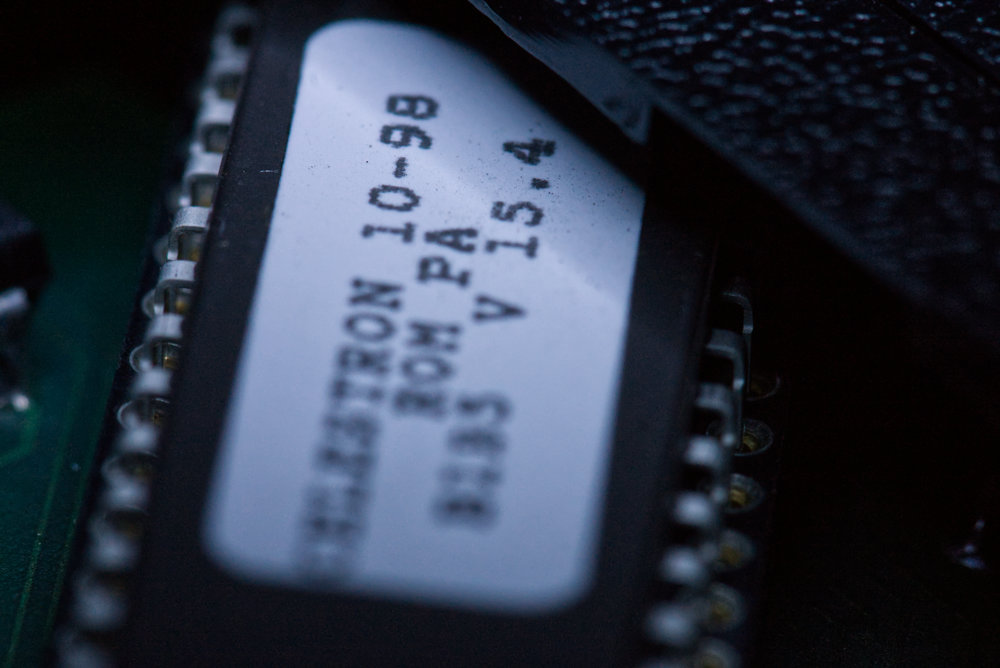The image is an extremely close-up and slightly blurred photograph of a black electronic device, presumably a computer chip or a part of a circuit board, sporting a white label with black text that is partially illegible. The visible text includes the fragmented sequences "TRON 10-98," and the second line reads "ROM PA." Further down, the text includes the series "B185 V 15.4," though some numbers are unclear. The label is situated in the center of the image, surrounded by a textured black component with metallic connectors. Gray metal conductors extend outward, leading into gold-accented holes. There are 14 visible clasps on the left and 8 on the right side of the label.